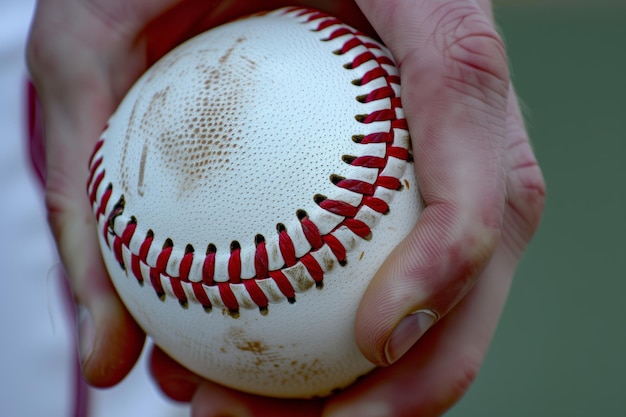In this highly detailed, close-up image, a person's taut hand grips a baseball with evident strain, highlighted by the purpling and reddening of their fingers. The hand appears slightly dirty, adding to the gritty realism of the scene. The baseball, off-white with distinct red stitching, shows scuffs and dirt marks that accentuate its aged texture. The stitching runs in a U-shape along the ball's surface, with visible tiny holes for the maroon threads. The person's four fingers are precisely positioned: one finger on the center, others on the back, and the thumb on the back left. Their worn fingers, with visible thin peach fuzz hairs, hint at a seasoned player. The background features a blurred dichotomy of green on the right, possibly a field or wall, and white on the left with indistinct details, possibly part of the person's clothing adorned with a red line.